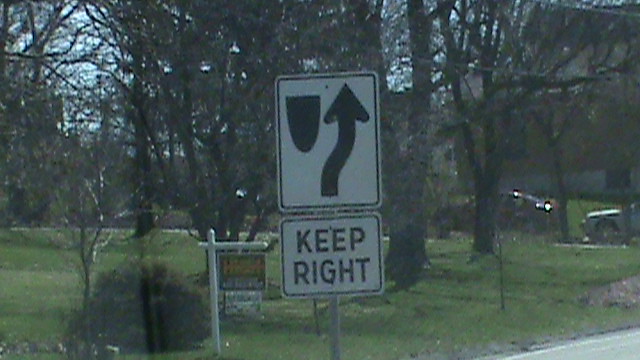This close-up photograph captures a detailed view of a roadside sign. The central focal point is a rectangular white sign, bordered neatly along the inner edge with a black outline. In the upper left corner of the sign, a bold, solid black "U" stands prominently. To the right of the "U," an upward-pointing arrow directs attention skyward, with its stem curling gently to the left at the base. Just below this, another white sign, also outlined in black, bears the simple, clear message "KEEP RIGHT" in black lettering. The signs are mounted on a silver pole, which extends downward and merges into a patch of vibrant green grass.

Surrounding the sign, the scene is set within a grassy area, dotted with trees in varying stages of foliage—some lush and leafy, others bare, exposing their branches. To the right and slightly behind the sign, a parking area is visible, with several parked cars, including a noticeable red vehicle in the middle right section of the photograph. In the lower left corner, a dark-leaved bush adds a touch of natural contrast against the bright green grass that dominates the foreground.